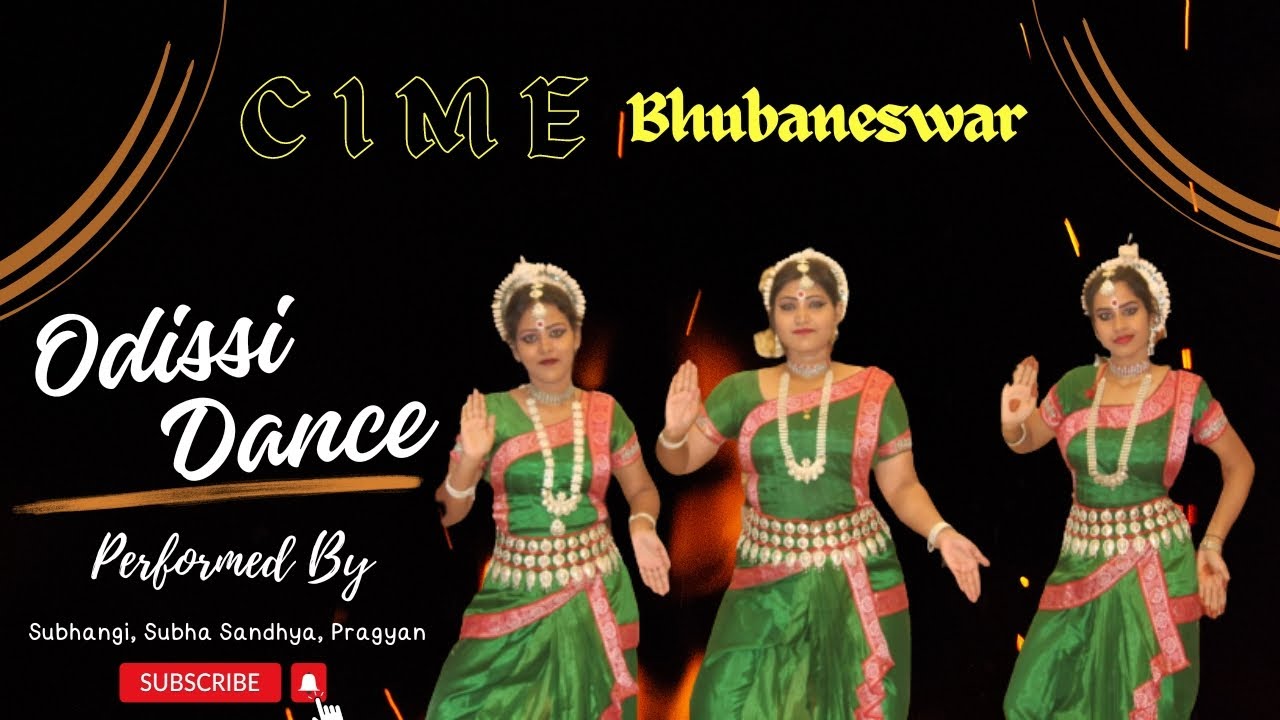The image is a vibrant advertisement featuring three Indian women in their twenties, prominently positioned in the foreground, dressed in matching green dresses with white headpieces and intricate white or silver necklaces. They are posed gracefully, with their right hands raised to display their palms and their left hands extended near their waists, also exposing their palms. The women, who have dark skin, dark eyes, and are adorned with red lipstick and wrist bangles, appear to be showcasing a traditional dance form.

Text overlays the black background of the image. Across the top, in bold yellow letters, is "CIME BHUBANESWAR." On the right side, written in elegant white script, is "ODISSI DANCE," followed by "performed by," and the names "SUBHANGI, SUBHASANDHYA, and PRAGYAN." This carefully composed image, likely a screen capture from a video, includes iconic YouTube elements such as a subscribe button and a notification bell, indicating that viewers can subscribe to receive updates on new performances. The overall arrangement suggests that this is promotional material for the dance group's video content.